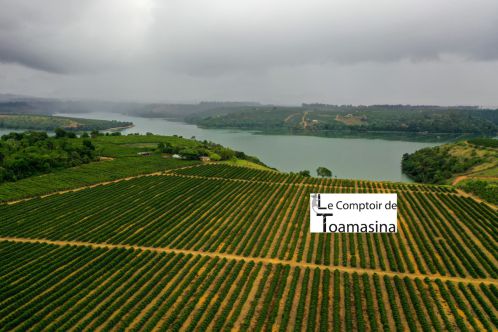This aerial photograph captures a lush, orderly farmland perched high above a serene body of water, surrounded by an expanse of green fields and dense forests. The meticulously cultivated crop rows are uniformly green, with vertical rows dominating the landscape and smaller horizontal paths interspersed for walking. The farmland takes up about half of the image, transitioning into a vibrant green backdrop of trees and grass on both the left and right sides. In the middle-right of the image, a notable logo, "Le Compteur de Tomasina," appears prominently in black text on a white background, perhaps resembling a label. The scene is enveloped by an overcast sky, heavily laden with dark gray clouds, hinting at imminent rain. The water below mirrors the somber tones of the sky, enhancing the tranquil yet moody atmosphere of this verdant and meticulously organized agricultural vista.